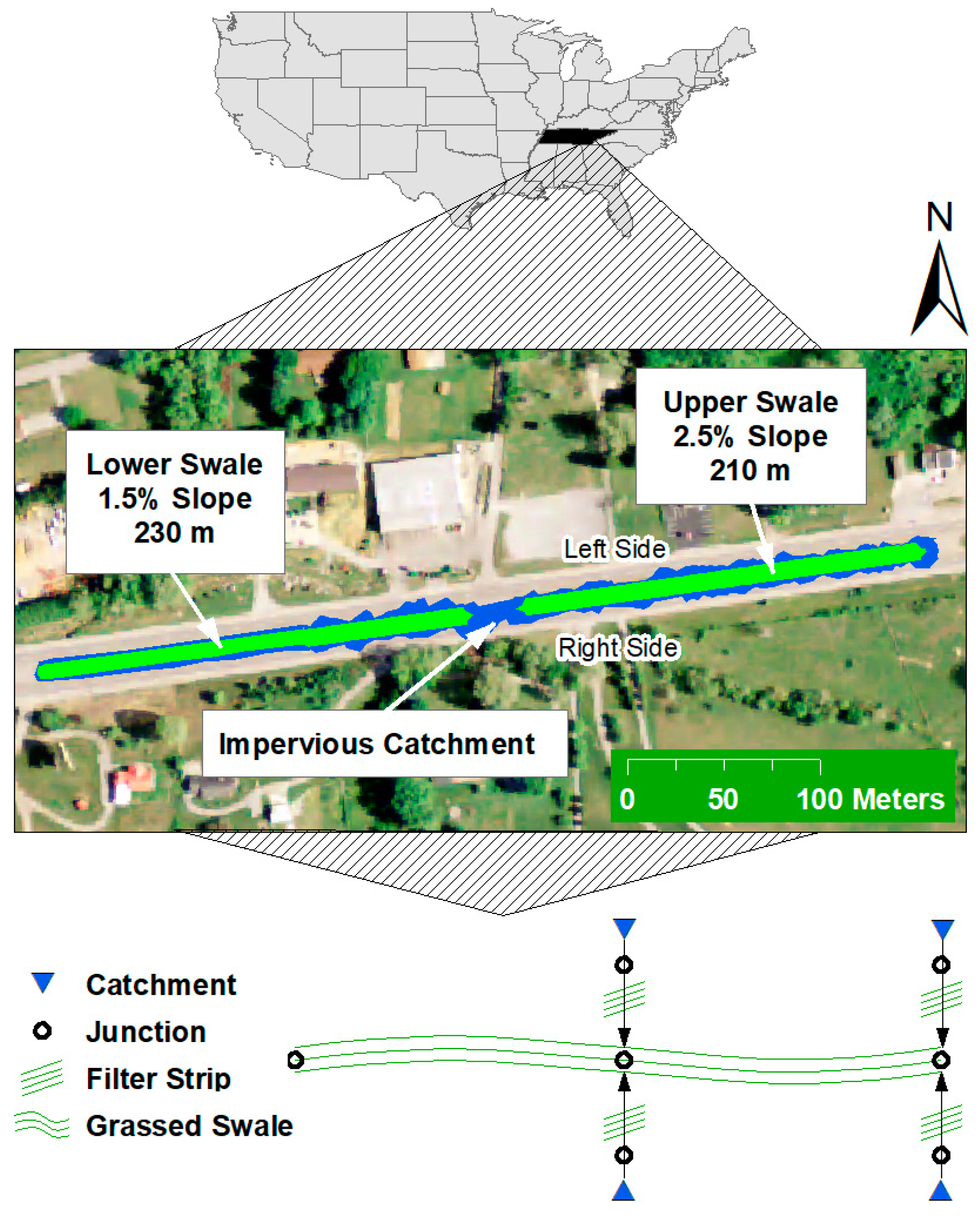The image is a detailed annotated map of a region in Tennessee. At the top, there is a small gray map of the United States with Tennessee shaded in black, highlighted by a connecting triangle pointing to a zoomed-in section below. This central section features an aerial view of a neighborhood in Tennessee, displaying homes, trees, grass, and driveways in natural colors. The image incorporates detailed topographical information, indicating areas with a lower swale of 1.5% slope extending 230 meters, and an upper swale of 2.5% slope covering 210 meters. These swales are marked as "impervious catchments" within the image. At the very bottom, there is a key with symbols: a blue chevron indicating 'catchment,' alongside other symbols representing a 'junction,' a 'filter strip' (three thin green lines), and a 'grassed swale' (three wavy lines). The illustration is further oriented by a compass arrow directing north in the bottom right corner.